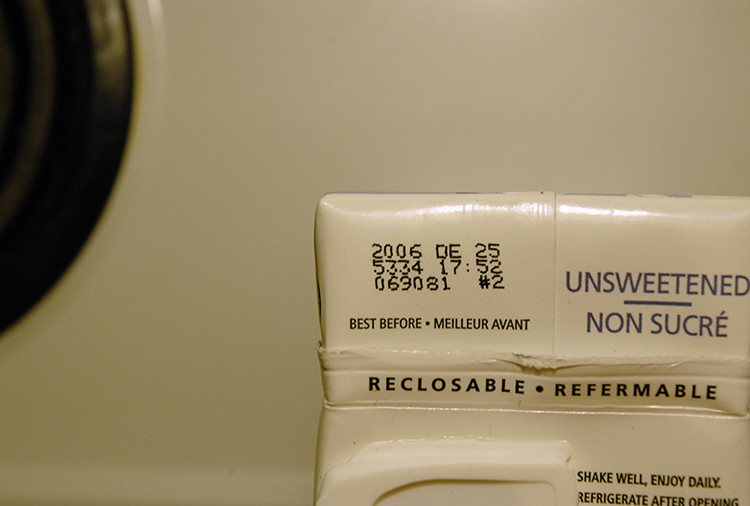The image captures the corner of a beige and black container, likely for juice or milk. The focus is centered on the 'Best Before' date, prominently displaying "2006 December 25th." Below the date, a time along with three lines of numbers are visible, possibly production details. On the right side of the container, the word "Unsweetened" is printed in blue, with "Non-sucre" in a smaller font underneath, indicating the content is unsweetened in both English and French. Along a seam, the phrases "Reclosable" and "Reformable" are printed in both languages. Near a spout designed for pouring, additional instructions are provided: "Shake well, enjoy daily, refrigerate after opening." The overall design appears functional and informative yet understated.